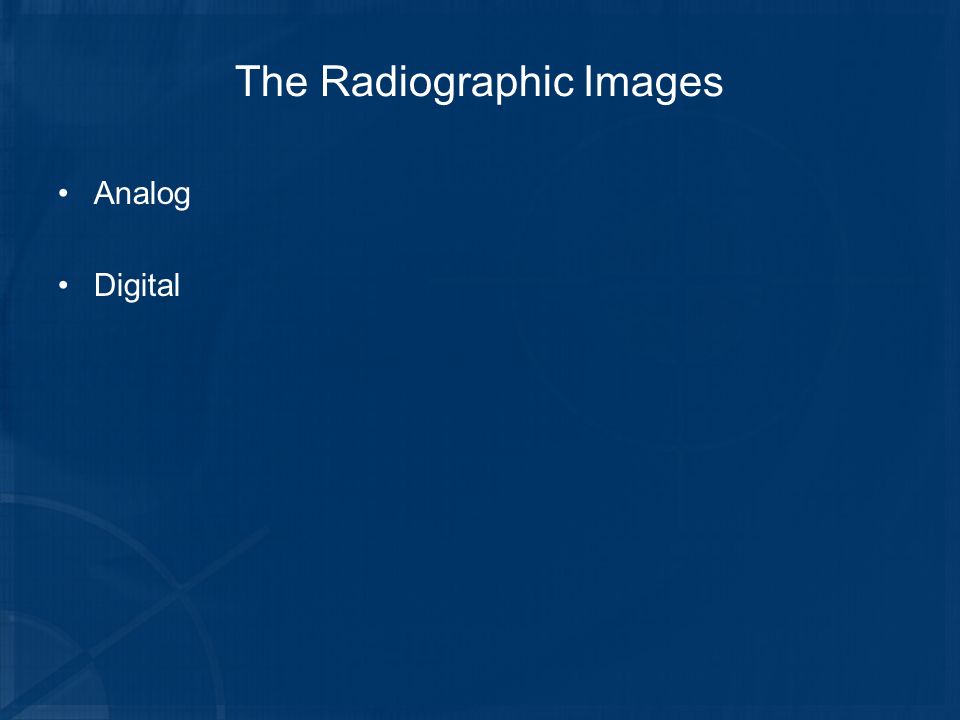This detailed square image features a navy blue PowerPoint slide with a simplistic yet informative design. At the top center, the title "The Radiographic Images" is displayed in white text with an initial capital letter for each word. The title is written in a plain font, consistent with the rest of the text on the slide. Beneath the title, on the upper left-hand side, are two bullet points. The first bullet point, marked by a small white circle, reads "Analog" with a capital 'A.' Directly below, the second bullet point, similarly marked, reads "Digital" with a capital 'D.' In the lower left corner of the slide, there is a subtle design element: a faint circular shape with a spear-like arrow piercing through it, reminiscent of a quarter compass rose, adding a touch of visual interest without detracting from the main content. All text is rendered in white against the dark background, ensuring clear readability.